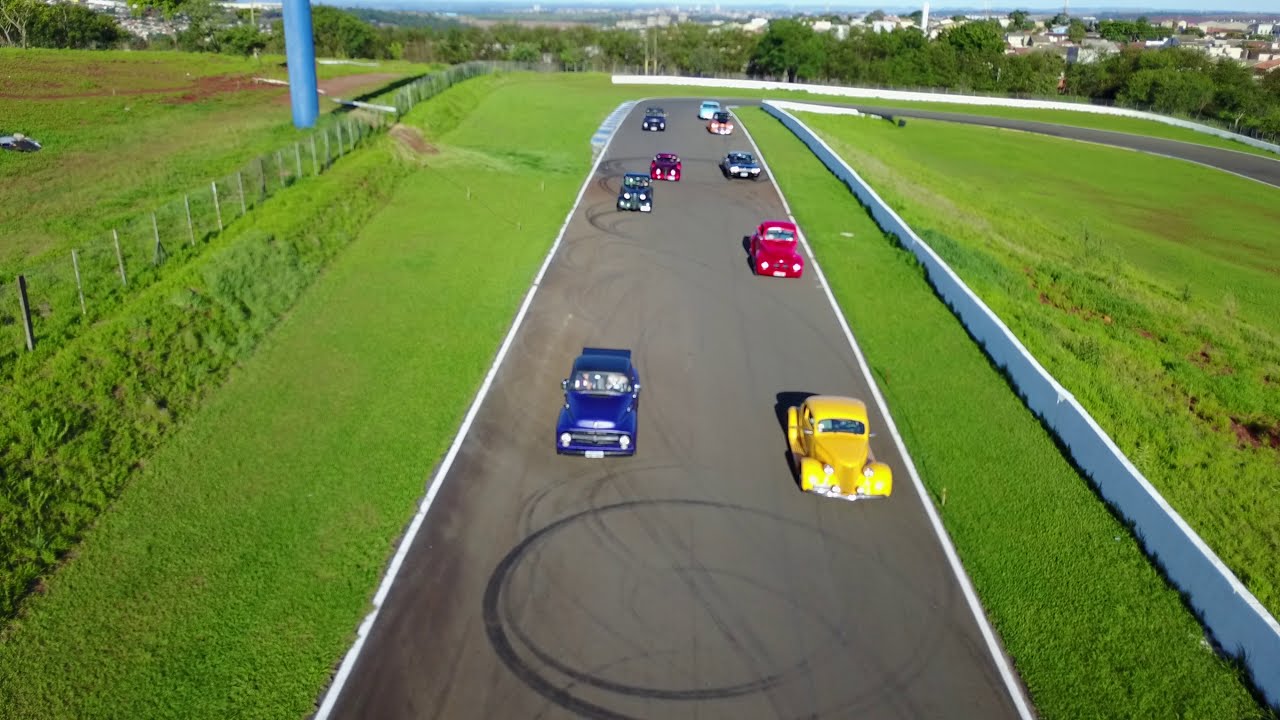This elevated photograph captures an exciting scene on a racetrack, showcasing a group of brightly colored vintage and antique cars poised for a race. The racetrack itself, gray and marked with tire patterns from previous maneuvers, including noticeable donut shapes, curves to the right midway through the image. There are nine cars in total, lined up and ready to go. Leading the pack on the inside track is a vibrant yellow car, often likened to a ZZ Top classic. Right beside it and slightly behind is a striking blue vehicle. Trailing these front-runners, there's an array of colorful cars including a red one, perhaps resembling a Mustang, a green Jeep, another red car, and further back, a silver Mercedes and a light teal car among others. Surrounding the track is a densely green grass-covered ground, mowed and well-kept, contrasting sharply with the gray asphalt. In the background, beyond the racetrack, lie buildings and trees, hinting at a nearby city or town. A white retaining wall runs vertically along the right side of the image from bottom right to the middle top, adding to the structural elements that frame this dynamic racing scene.